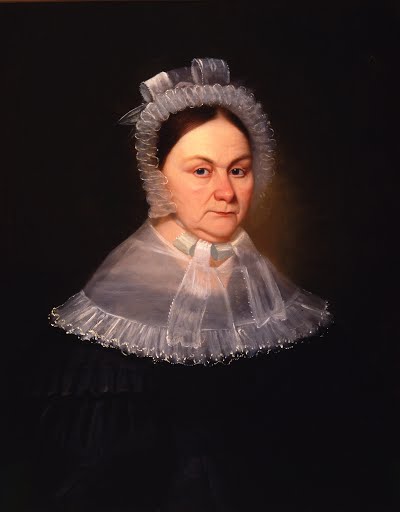The image is likely a photograph or an oil painting of an older woman from a past century, possibly the 18th or 19th. She appears to be in her 30s or 40s. The background of the image is predominantly black, with slight hints of light brown around her face, making her features stand out starkly against the dark backdrop. She has a serious, almost passive expression and gazes directly at the camera.

The woman wears a black dress that subtly blends into the dark background. Over her dress, she has draped a shawl made of a sheer, almost translucent material, potentially lace, that provides a glimpse of her skin and dress beneath it. Her head is adorned with a bonnet made of the same delicate, see-through fabric. The bonnet is tied with a ribbon under her chin, and additional ribbons at the top are tied into a bow behind her head. Her brown hair is slicked back to each side, and she has very fair skin and brown eyes. Notably, she wears no makeup, emphasizing the natural, unembellished look typical of the period depicted.